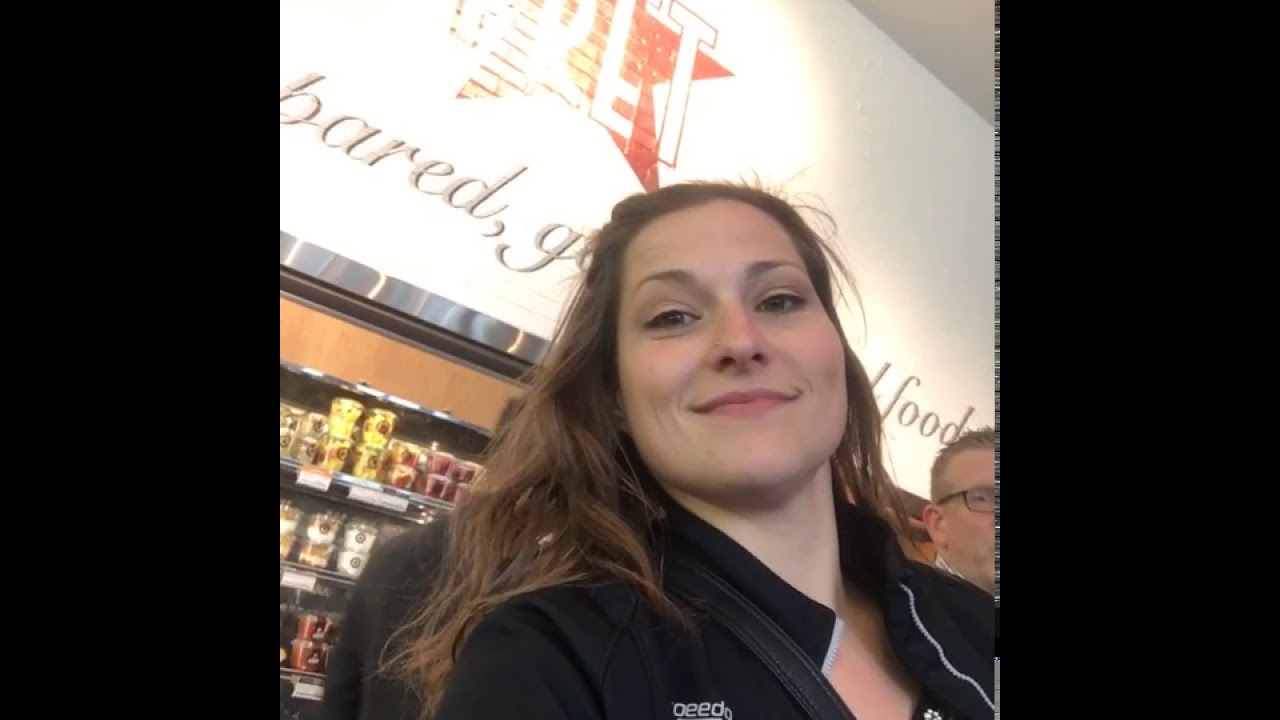This is a close-up selfie of a young Caucasian woman in her early 20s, standing inside a grocery store. She has light brown hair pulled back from her forehead, falling over her shoulders, and she is smiling into the camera. She is wearing a black jacket with white trim. The photo is framed from her chest up to her head, placing her at the center, slightly to the bottom right. Behind her, there is a wall with shelves stocked with various food products in plastic containers, displaying colors like red, yellow, and white. Above the shelves on the wall, there is a partially obscured script reading "B-A-R-E-D, G" and the word "F-O-O-D" to the right. Additionally, there's a store logo featuring a red star with horizontal stripes and possibly the letters "V-R-E-T" above it. Another noticeable detail in the background is half of a man's face with short light brown hair and dark-framed glasses, positioned in the bottom right corner.